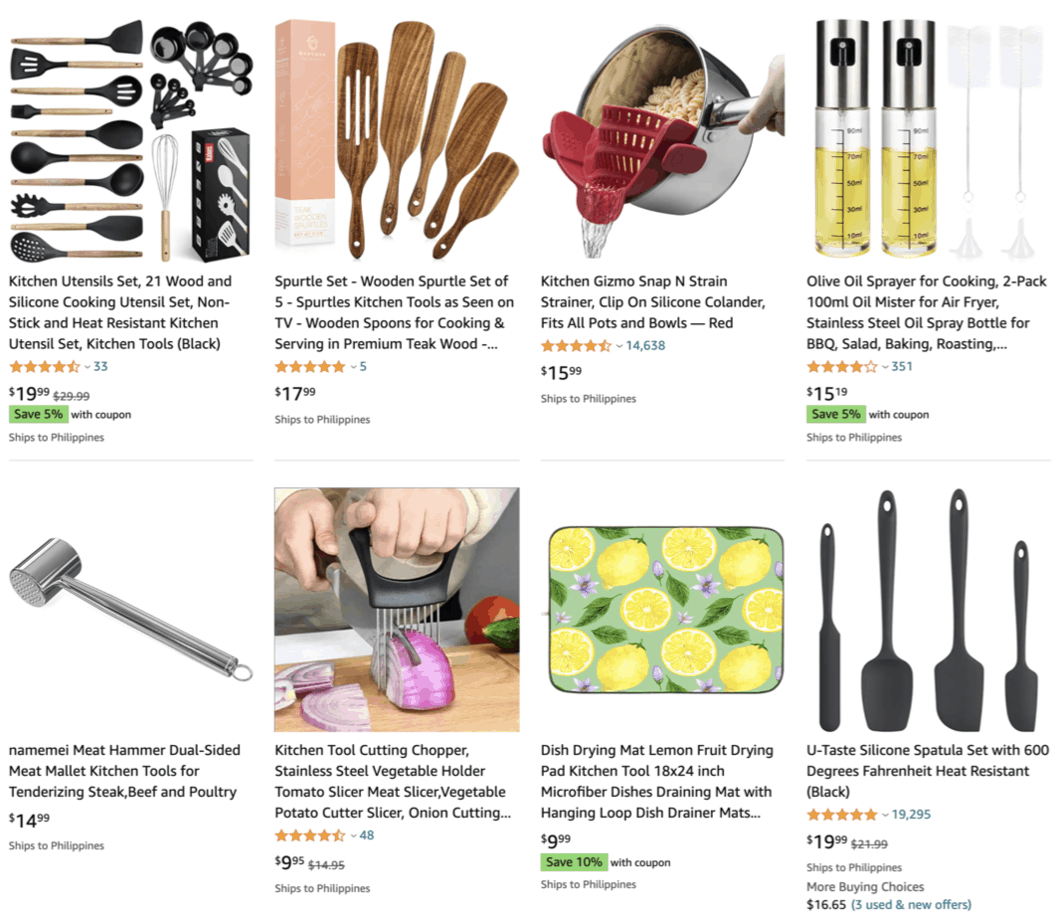This image depicts a cropped screenshot of an Amazon webpage showcasing eight different kitchen products arranged in two rows. The top row features a comprehensive kitchen utensil set that includes various spatulas, sieves, a whisk, and measuring spoons. Following this is a wooden spurtle set, comprising elongated paddle-like utensils called spurtles. Next is the Kitchen Gizmo Snap and Strain Strainer, which can be clipped onto pots to serve as an efficient straining device. The fourth item on the top row is an olive oil sprayer designed for cooking, packaged in a sleek bottle.

The bottom row begins with a robust meat hammer or mallet, essential for tenderizing meats. This is followed by a vegetable chopping device, designed to streamline the cutting process. Next is a dish drying mat, an absorbent surface to place wet dishes after washing. Lastly, there is a heat-resistant spatula set, ideal for various cooking tasks.

Each product is clearly displayed, offering a glimpse into their practical uses, emphasizing their utility in a modern kitchen.